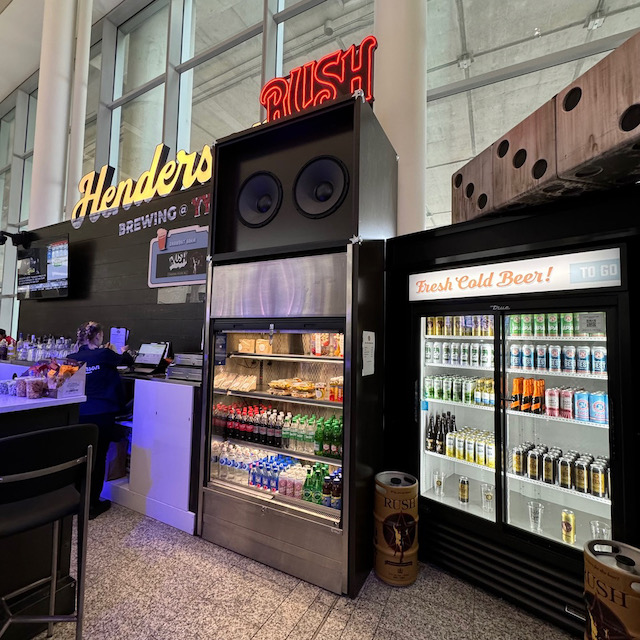This image captures a vibrant section of Henderson Brewing themed after the iconic rock band Rush, located in the Toronto Pearson International Airport (YYZ). Dominating the scene are two neon signs illuminating the words "Henderson" and "Rush," suspended above a tall fridge. On top of this fridge, there's an eye-catching, large speaker-like structure. Inside, a variety of snacks are displayed, while the lower section of the fridge offers an assortment of drink options.

To the right, another fridge labeled "Fresh Cold Beer To Go" stores an array of bottled and canned beverages, some adorned with Rush-themed labels. A slice of the bar counter is visible to the left, along with a bartending staff member attending to patrons. The setting exudes a modern, energetic vibe, merging the worlds of craft brewing and legendary rock music.

In the upper right corner, dice are depicted, a nod to Rush's "Roll the Bones" album, enhancing the thematic decor. At the bottom of the image, a collection of Rush-branded kegs is neatly arranged. A selection of Rush-themed beers is prominently featured within the "Cold Beer To Go" fridge, appealing to fans of both the band and craft beer aficionados.

The overall environment seamlessly blends elements of music, food, and craft beverages, presenting a lively homage to Rush within a contemporary brewery setting.